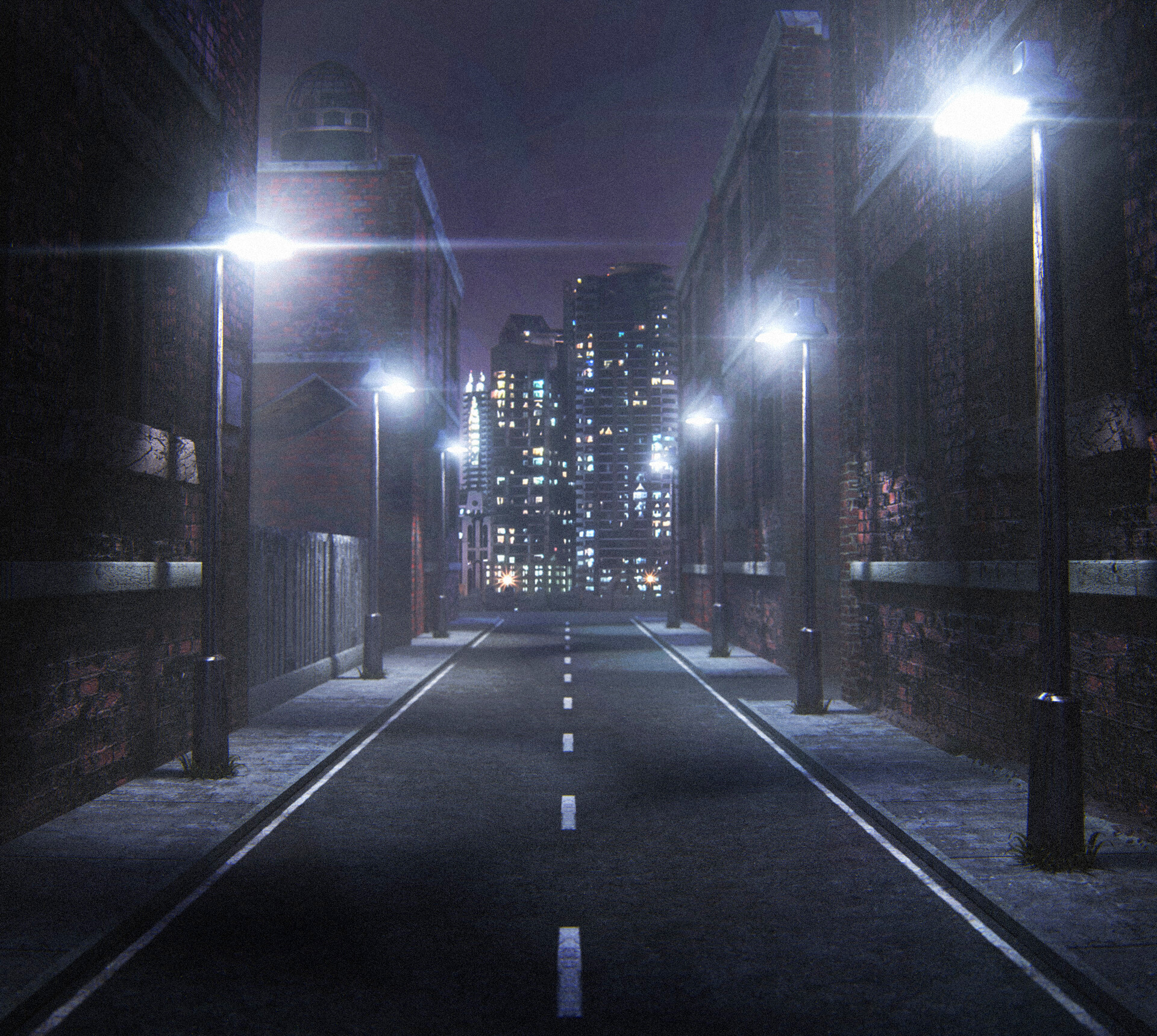This image, likely AI-generated due to its perfect alignment and spacing, depicts a serene city street at night. The dark black asphalt pavement, marked by white lines on either side and a dashed white line down the center, extends into the distance. Tall black streetlights, evenly spaced on both sides of the road, cast bright pools of light onto the scene. The left side has three streetlights, while the right side features four. Flanking the street are low, two-story brick buildings with gray stone sidewalks that lack parking spaces. On the left side, a fence separates two of the buildings, adding a touch of variance to the architecture. In the background, two towering business buildings, approximately 30 to 40 stories high, loom over the street. These buildings are adorned with a grid-like pattern of windows, each illuminated with lights of varying colors including yellow, light blue, white, and orange, contrasting against the night sky. The street is notably devoid of vehicles and pedestrians, emphasizing the stillness and order of this urban landscape.